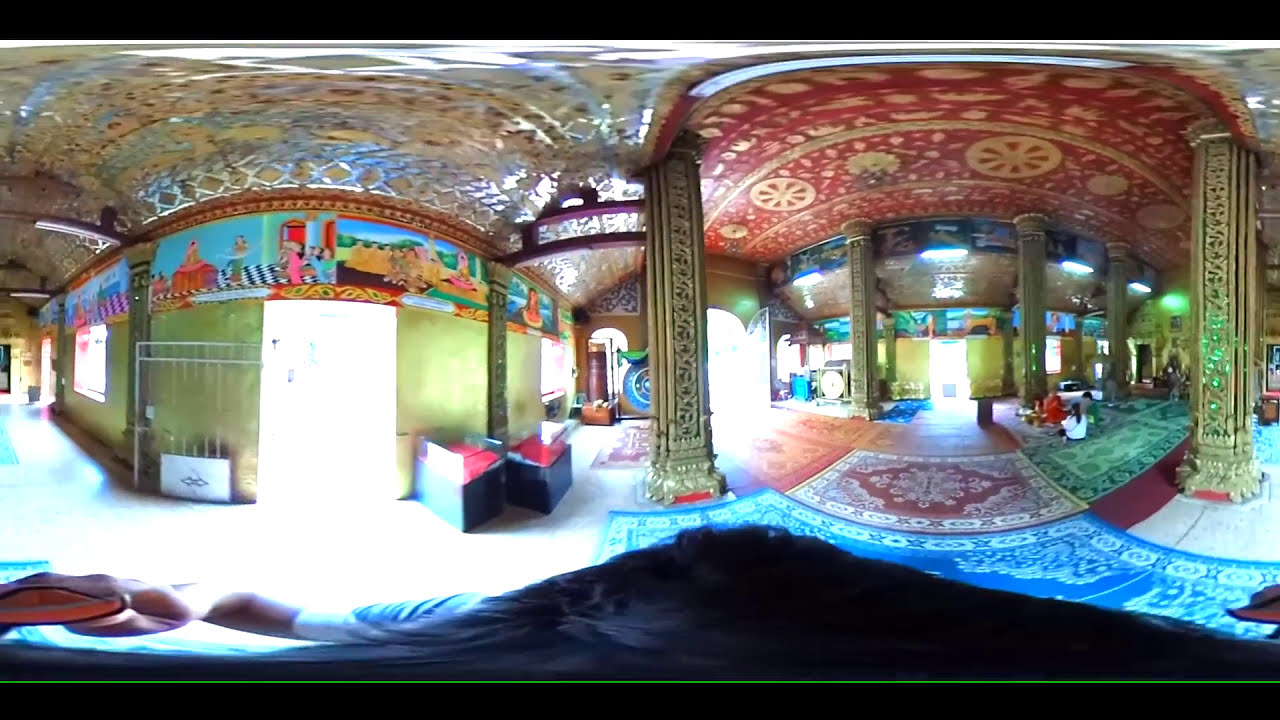This image depicts the vibrant interior of a religious building, possibly a mosque or an Indian temple, captured in a squashed 360-degree panoramic format, creating a distinct distortion. The brightly lit space is adorned with a rich tapestry of colors including red, blue, green, and gold that are prominent throughout the decor. The ceiling is elaborately designed with colorful geometric patterns and intricate frescoes. The walls showcase traditional art, including murals depicting various scenes, such as individuals in buildings, fortresses, and riding elephants.

The floor displays an array of colorful carpets and several multicolored rocks, adding to the traditional aesthetic. Ornate, filigreed pillars are found throughout, with at least four square-designed columns featuring elaborate patterns. The interior space also includes multiple doorways and windows letting in an abundance of sunlight. In the right-hand corner, people are seated cross-legged on rugs, appearing to be in prayer or meditation, contributing to the serene atmosphere. Additional elements, such as gongs and other religious artifacts, are also present within the space.

The image appears to be taken from above, perhaps from a head-mounted device, given the visible hands and distortion suggesting a fisheye lens effect. This unique vantage point, coupled with the vivid and diverse array of colors and intricate designs, encapsulates the essence and beauty of this sacred interior space.